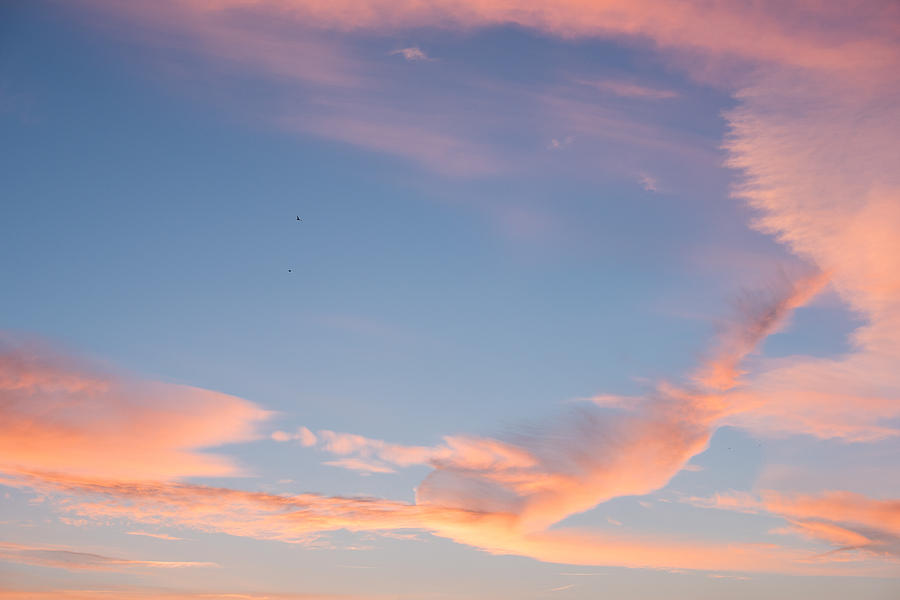The image depicts a serene, peaceful sky at sunset, characterized by a stunning array of colors. Against a backdrop of open blue sky, thin wispy clouds, heavily tinted with shades of pink, red, and orange, stretch across the scene, giving the impression of a painterly cotton candy effect. The thicker, bolder clouds are primarily positioned at the bottom and right side of the image, while the center and top left corner remain clear, adding to the tranquil feel. The scene is punctuated by two tiny birds, flying in the distance near the center-left part of the image. The blending hues and the absence of any other elements like planes or buildings create a harmonious and undisturbed atmosphere, perfect for capturing the tranquil essence of a setting sun.